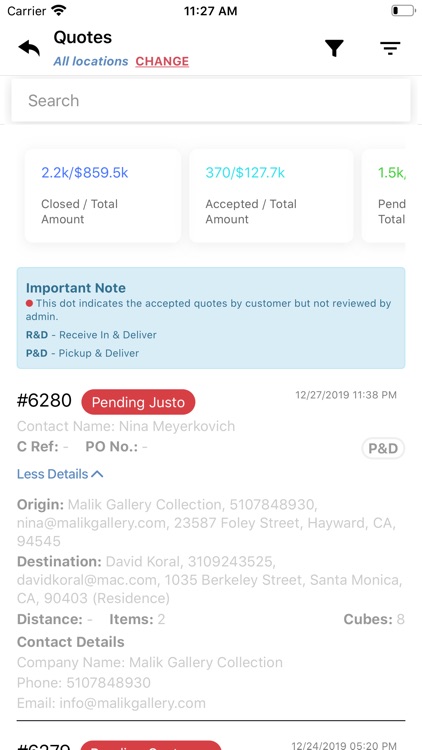The image is a screenshot from a cell phone displaying a detailed interface on a white background. In the top-left corner, terms like "carrier" and the Wi-Fi symbol are visible. The center shows "11:27 AM," while the right-hand side displays the battery icon with a low battery level. There is also a black status bar present.

In the main content area:
- The word "quotes" is in black letters.
- A black left arrow is also visible.
- Beneath, the phrase "all locations" is marked in blue.
- The word "CHANGES" is highlighted in uppercase red letters with an underline.
- A search box is included.

Below the search box, three different status boxes provide detailed metrics:
1. **First Box**: Blue with white text stating "2.2K / 859.5K closed / total amount".
2. **Second Box**: Blue with white text saying "370 / $127.7K accepted / total amount".
3. **Third Box**: Partially visible, displaying "1.5K,...".

Next, a blue rectangular box titled "IMPORTANT NOTE" is accompanied by a red dot. The note explains that the red dot indicates quotes accepted by the customer but not reviewed by admin. It mentions R&D/receive in and deliver, and P&D/pick up and deliver.

Following this note:
- The black number "6280" is displayed.
- A small red bubble labeled "pending JUSTO" is alongside.
- Date and time "12/27/2019, 11:38 PM" are shown.

Further details listed include:
- CREF Number
- Origin
- Destination
- Distance
- Items (2)
- Cubes (8)
- Contact details comprising the company name "Malik Gallery Collection," a phone number, and an email address.

The intricate details in the image suggest it is of a complex software interface possibly related to logistics or transportation.